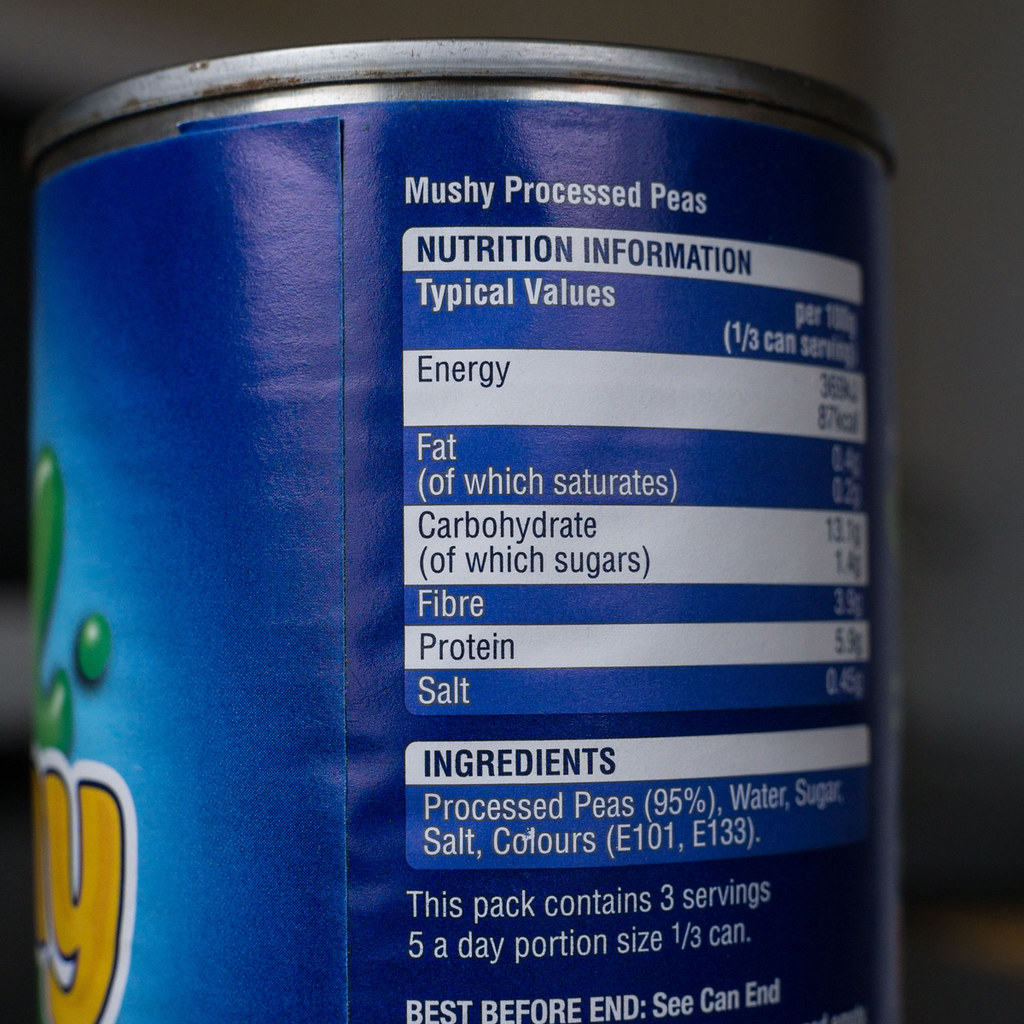A close-up image showcasing the nutritional information for a can of mushy processed peas. The can is silver, prominently featuring a blue label on its left side. The label displays a green, indiscernible blob and a yellow 'Y' set against a white background. The detailed nutritional information is organized alternately between white text on a blue background and blue text on a white background, presenting values for energy, fat, carbohydrates, fiber, protein, and salt. The ingredients include processed peas, water, sugar, salt, and colors. The label indicates that the can contains three servings, contributing to a "five a day" portion size of one-third of a can. Additionally, the "best before end" date is advised to be checked on the can itself.